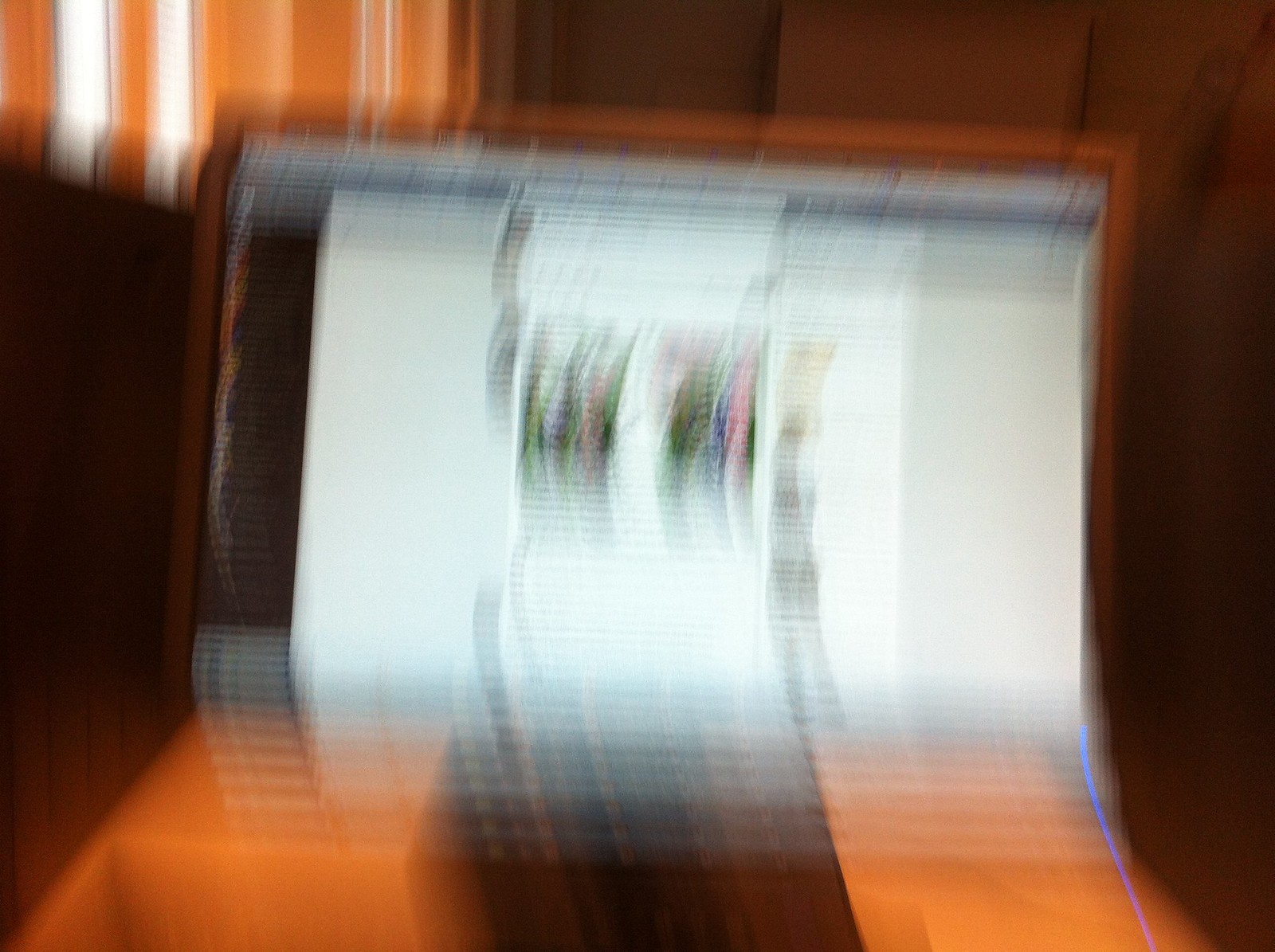The image depicts a highly blurred photograph, centered around what appears to be a silver computer monitor on a wooden desk or wall unit. The monitor screen features a dominant white rectangular shape, possibly displaying smaller images or photographs against a white background. In front of the monitor, there are two gold rectangular objects, offering a contrast with their distinguishable light and dark shading, though their precise nature is unclear. The background reveals wooden paneling on the right, adding a rustic touch to the setting. In the upper left corner, a window shade in shades of light brown and cream is partially visible, pulled down to cover the window. The overall image is quite unclear, making it challenging to discern finer details.